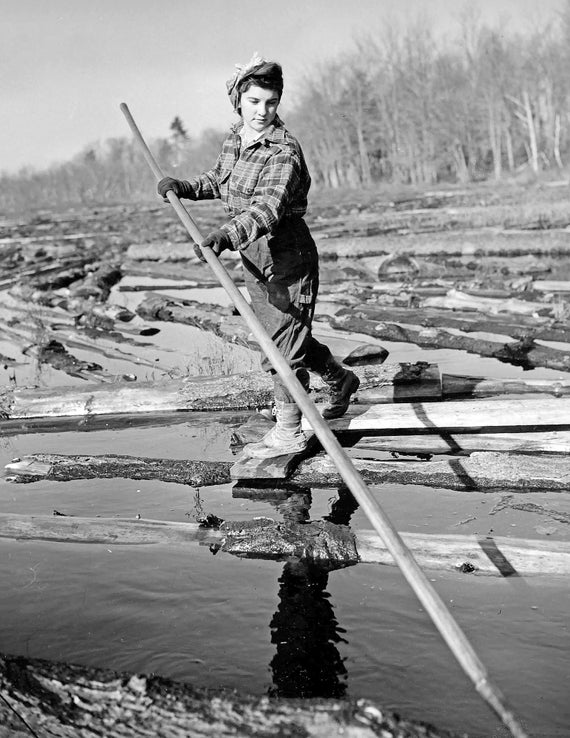This is a detailed, vintage black-and-white photograph from the 1930s or 1940s, showcasing a woman working in the logging industry, most likely during the war period. The image captures her amidst a wide river filled with floating logs, as she skillfully employs a very long pole to break up logjams, ensuring smooth transportation down the river. She balances adeptly on adjacent logs, highlighting her expertise in this arduous task. Dressed in deep waders, a flannel shirt, gloves, and with her hair tied in a bandana, she stands confidently in a forested area marked by both cut and standing trees along the riverbanks. Her attire and the scene suggest the demanding nature of her work, with the backdrop of numerous logs emphasizing the scale of this logging operation.